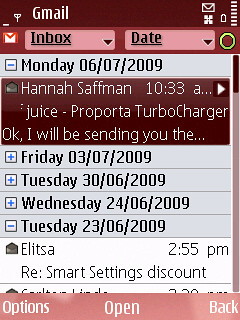This image is a rectangular screenshot taken from a phone displaying a user’s Gmail account. At the top, a maroon horizontal rectangle features the white text "Gmail" in the left-hand corner. Below this, there are two pink rectangles labeled "Inbox" and "Date," each with a black arrow pointing downwards indicating clickable options. Adjacent to these labels, there is a small green circle. 

Underneath, a row with a gray background shows the date "Monday 06/07/2009." Beneath this date, a maroon rectangle includes the text "Ahana Safman," with the time "10:33 AM" and a cryptic snippet of the email content mentioning “Juice, Proporta, Turbocharger, OK, I will be sending you the.” Below this, gray rows list additional dates and email previews. Another distinct email is marked "Tuesday 23/06/2009" from "Elitsa" concerning "smart settings discount."

At the bottom of the screenshot, typical navigation options such as "options," "open," and "back" allow the user to move through the Gmail interface efficiently.